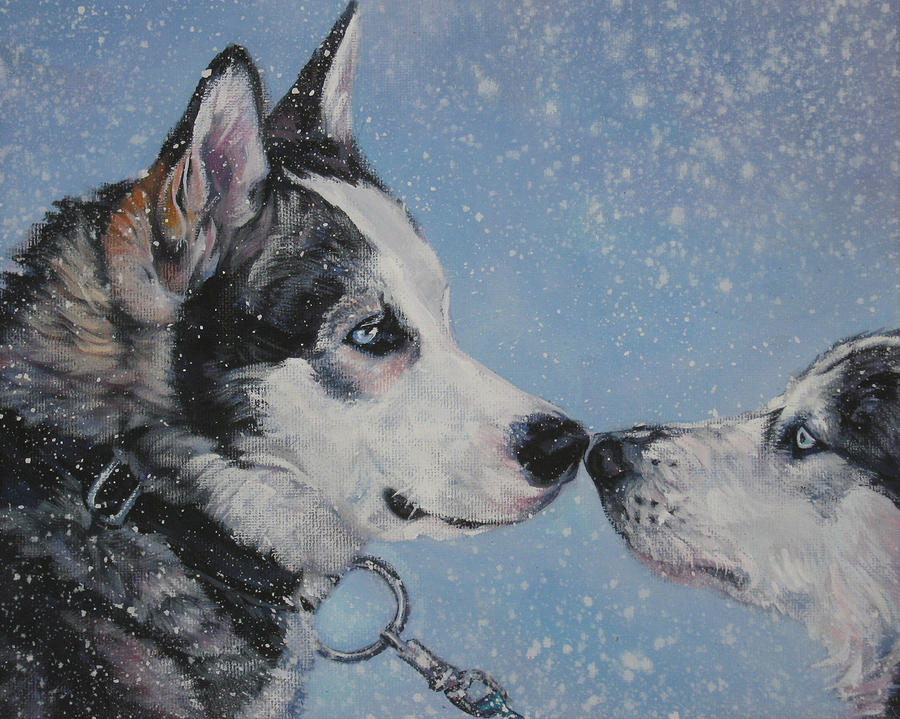This image depicts an oil painting of two Alaskan Huskies pressing their noses together, creating an intimate and captivating scene. The background features a light blue, grayish sky with heavy snow falling, contributing to a somewhat gloomy yet serene atmosphere. The dog on the left has its entire head, neck, and shoulder visible, sporting a predominantly white face, dark gray head, back, and shoulders, with a distinctive reddish-orange hue around its ears. It wears a black collar with a prominent silver metal ring and a clasped leash attached to it. Both dogs have striking pale blue eyes, enhancing their soulful gaze as they touch noses and appear to look into each other's eyes. The dog on the right, positioned slightly lower, is partially visible from its nose to just behind its eyes, presenting a white-faced, gray-headed appearance. The texture of the canvas is apparent, emphasizing the detailed and artistic nature of the painting.